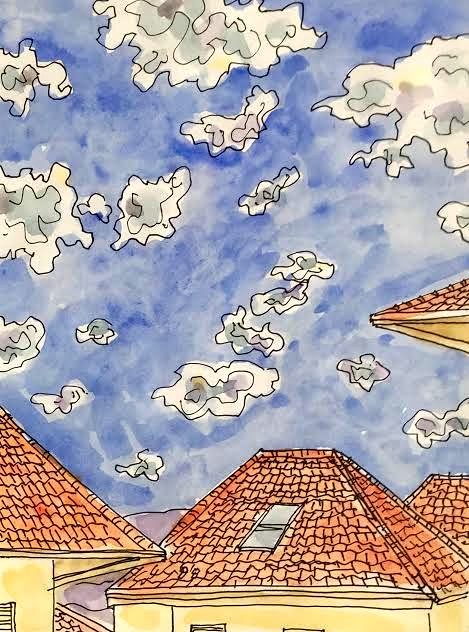This image depicts a vibrant, cartoonish painting showcasing a quaint rooftop scene. The roofs, characterized by their hip structure, boast a textured, orange-tiled appearance, adding warmth and charm. Each roof features a skylight, portraying small windows that hint at the life within. Above, a brilliant blue sky with scattered white clouds stretches expansively, contributing to the serene atmosphere. The exterior walls of the buildings are painted in a plain yellow hue, suggesting a material like concrete, EIFS, or stucco, though the precise texture is indistinguishable. The composition primarily focuses upwards, drawing attention to the harmonious blend of architectural elements and the picturesque sky.